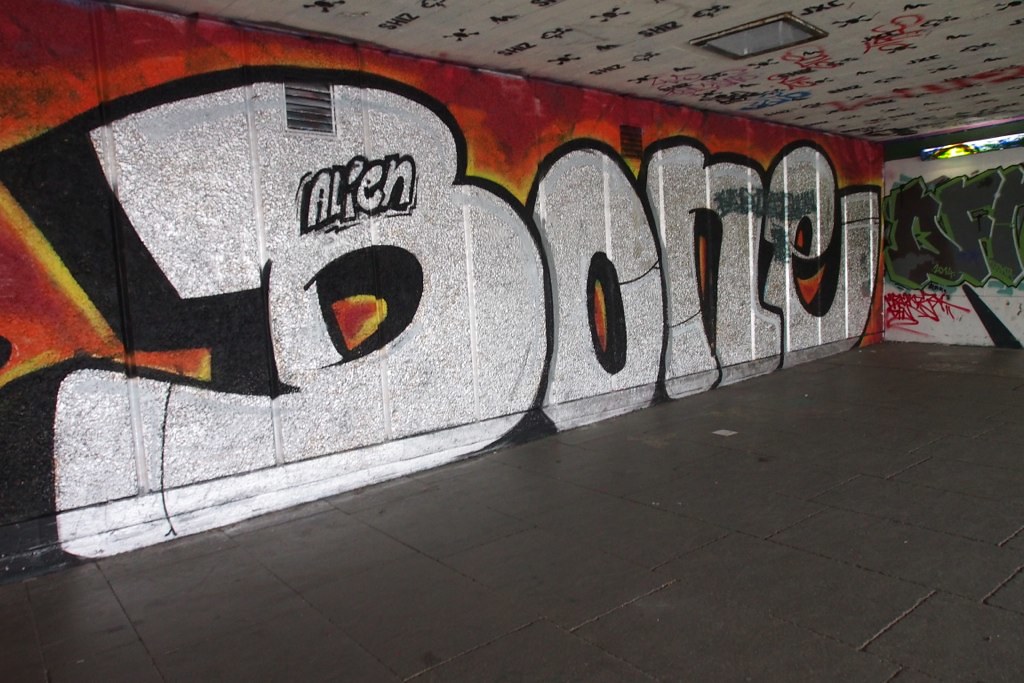This photograph captures an indoor scene featuring an extensive graffiti mural spanning a wall. The main wall, approximately 30 to 40 feet long and 12 to 15 feet high, is adorned with large, stylized white letters spelling out "BONE" with black shadows. Intriguingly, within the letter "B," the word "alien" is inscribed. The background of the wall displays a vibrant combination of deep orange, reddish, and yellow hues. The room itself appears to be well-maintained, suggesting the graffiti might be an intentional artistic installation. The floor is covered with dark square tiles, and the ceiling is white, hosting numerous logos and a light socket without an active light. Adjacent to the main wall is a perpendicular white wall featuring illegible green and red graffiti, adding to the eclectic atmosphere of the space.